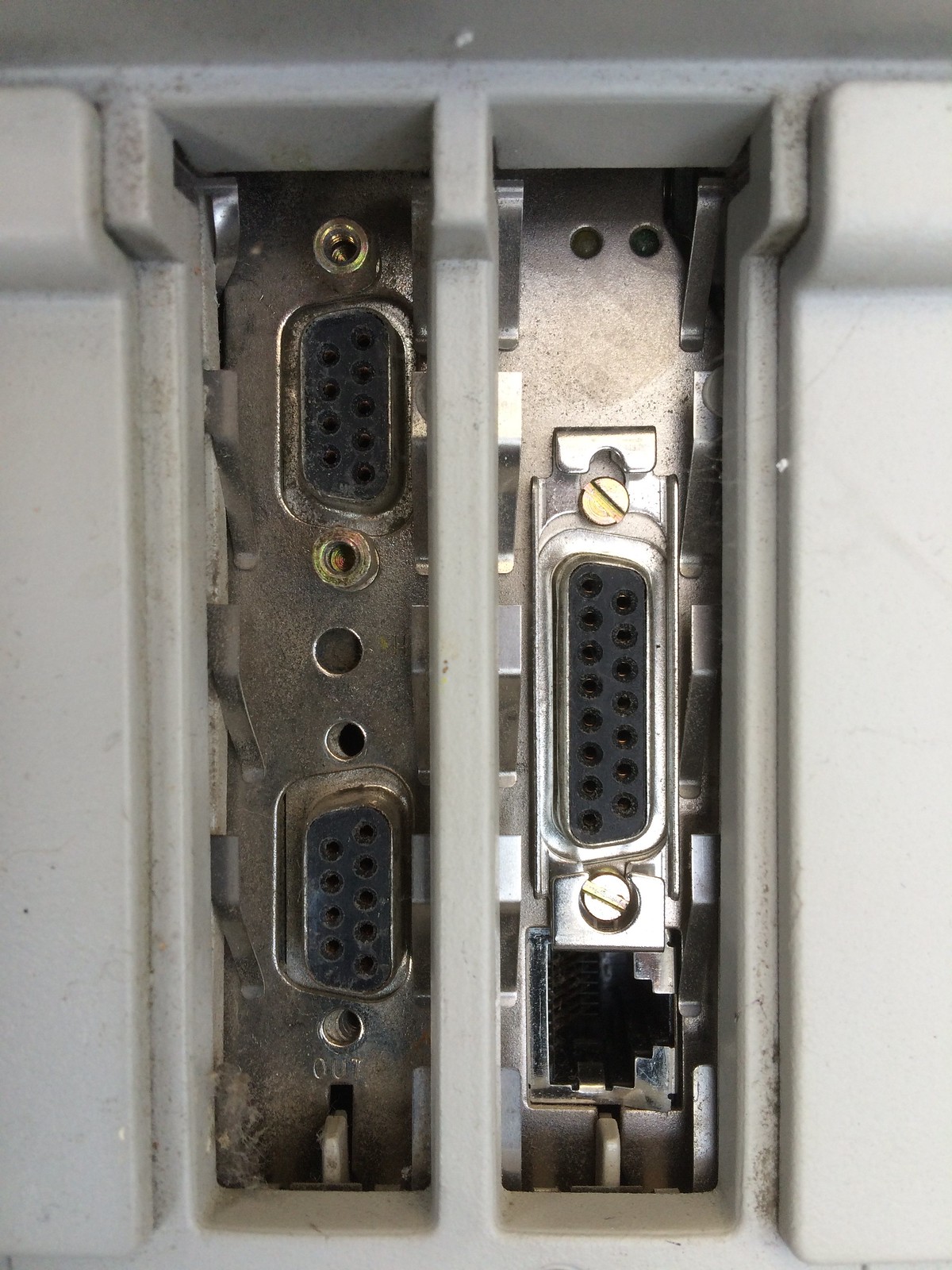The image shows the rear panel of a metallic-colored electronic device, possibly a computer or a monitor. The panel features several input connectors, specifically VGA ports. On the left side, there are two smaller, rectangular connectors, each with nine pinholes. These are separated by a larger gap with additional mounting holes. On the right side is a single, longer connector featuring 15 pinholes. The connectors are secured in place with black inserts and metal screws on the sides. The entire assembly is enclosed in a gray, square compartment, without any text or labeling.